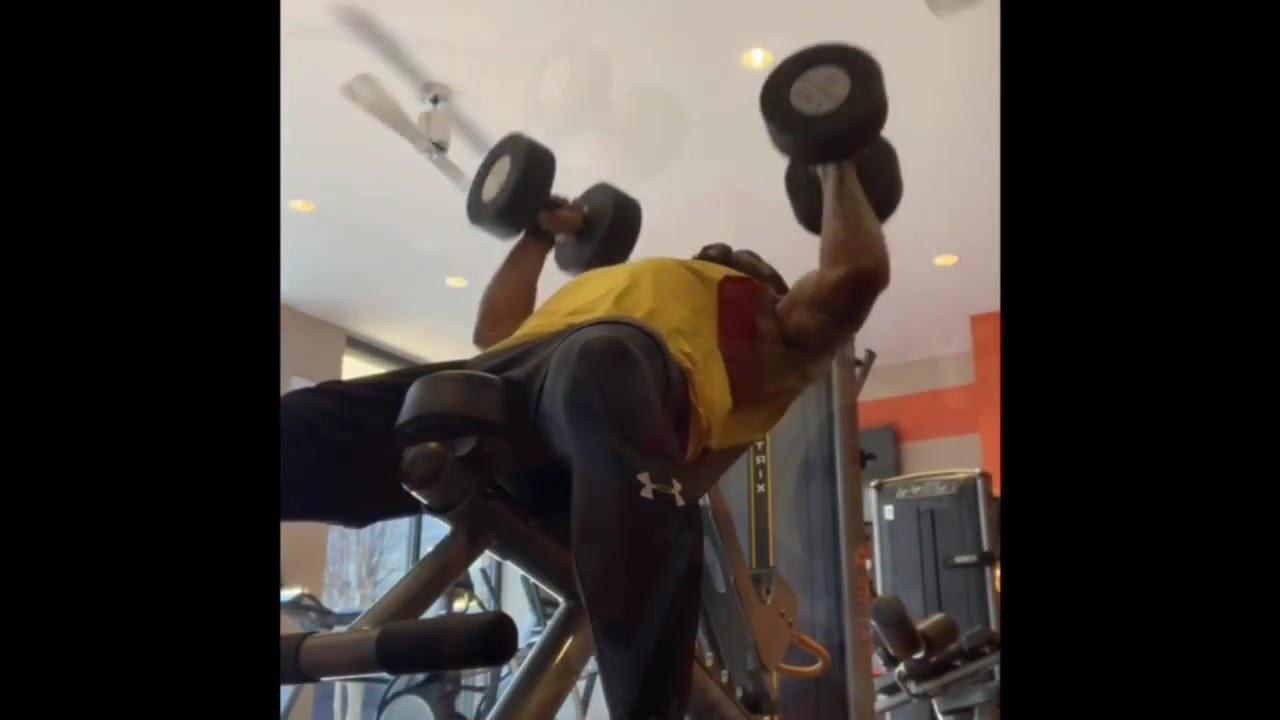The image depicts a very muscular black gentleman working out in a brightly lit gym during the daytime. He is positioned on an inclined weight bench, holding up large, black circular dumbbells with gray handles in both hands. He is dressed in black Under Armour leggings and a yellow tank top layered over a red shirt. His knees are facing the viewer, and he is leaning back with arms bent, showcasing his strength. Although his face is not visible, he appears to have short hair and possibly a beard. The gym has white ceilings with recessed lights and a ceiling fan, along with tan and orange walls adorned with additional weight equipment. In the background, a three-paneled window and a sliding glass door reveal daylight and blue skies outside.